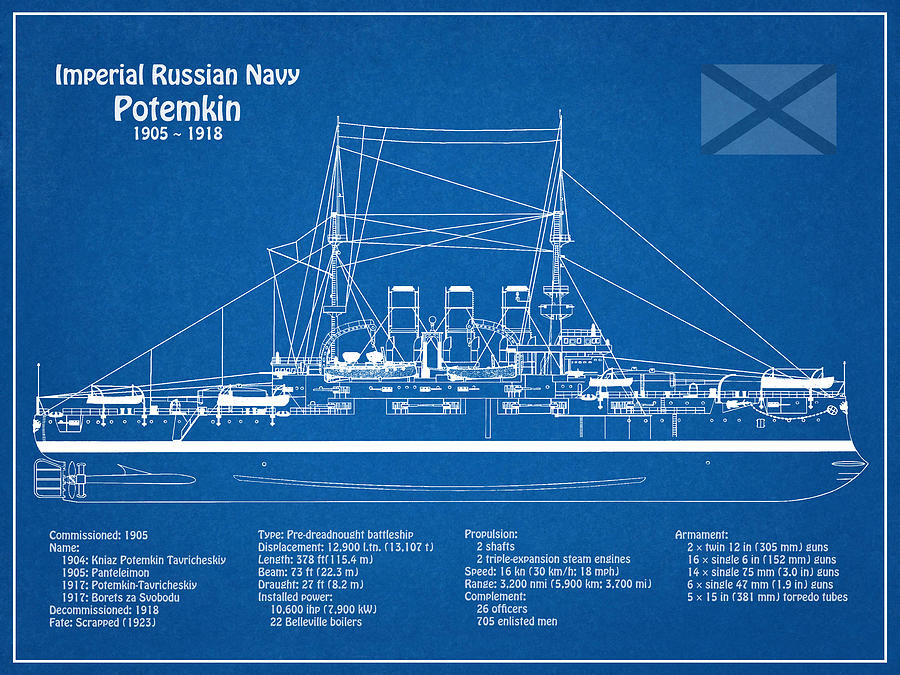This image is a blueprint-style diagram of the Imperial Russian Navy battleship Potemkin, active from 1905 to 1918, with a blue background and white text and lines. In the top left corner, it reads "Imperial Russian Navy" followed by "Potemkin" and the years "1905 to 1918". The side view of the ship spans the center of the image, displaying details such as two masts, three steam pipes centrally located, lifeboats, portholes, and propellers at the back. The diagram separates the above-water and below-water sections of the vessel with fine detailing along the deck. A white rectangle with black stripes forming an X is positioned in the upper right, possibly a flag or stamp.

Along the bottom, four columns of text provide comprehensive information about the ship. The first column states the ship's commissioning in 1905, and various renamings between 1904 and 1917, followed by its decommissioning in 1918 and scrapping in 1923. The second column describes the ship type as a pre-dreadnought battleship with a displacement of approximately 12,900 tons, a length of 378 feet (115.4 meters), a beam of 73 feet (22.3 meters), and a draft of 27 feet (8.2 meters). Its installed power was 10,600 horsepower (7,900 kilowatts) with 22 Belleville boilers. The third column lists the propulsion system as two shafts with two triple-expansion steam engines, allowing a speed of 16 knots (30 km/h or 18 mph) and a range of 3,200 nautical miles (5,900 km or 3,700 miles). The ship’s complement included 26 officers and 705 enlisted men. The fourth column details the armament: 2 twin 12-inch (305 mm) guns, 16 single 6-inch (152 mm) guns, 14 single 75 mm (3-inch) guns, 6 single 47 mm (1.9-inch) guns, and 5 torpedo tubes of 15 inches (381 mm).